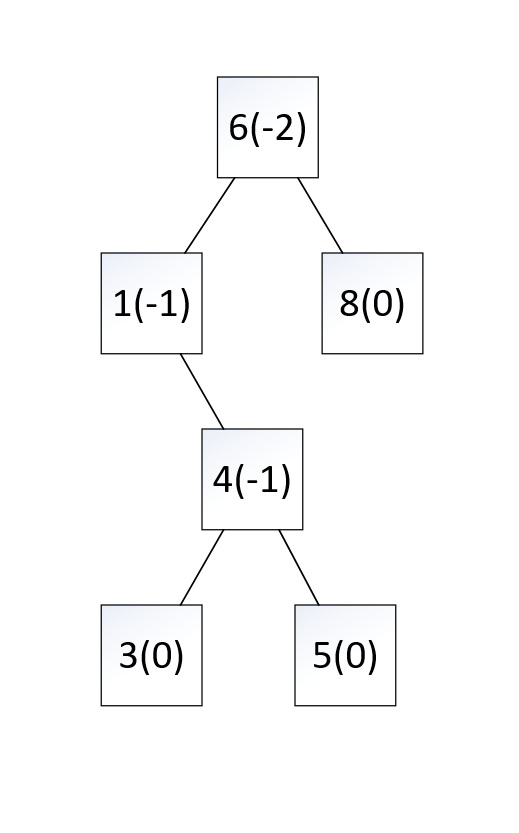The image depicts a flowchart against a white background featuring six interconnected boxes outlined in thin black borders. At the top center, the primary box contains the expression "6(-2)". Two lines descend from the bottom of this box in a V-shape, branching off to connect with two lower boxes.

The box connected by the right-angled line houses the expression "8(0)". Conversely, the left-angled line attaches to a box labeled "1(-1)". From this "1(-1)" box, a line extends downward to the right, leading to another box labeled "4(-1)".

From the "4(-1)" box, two lines extend downwards. The leftward line connects to a box that contains the expression "3(0)", while the rightward line connects to a box labeled "5(0)". Each of these interconnected boxes presents a distinct numerical and parenthetical expression, creating a structured and detailed flowchart.